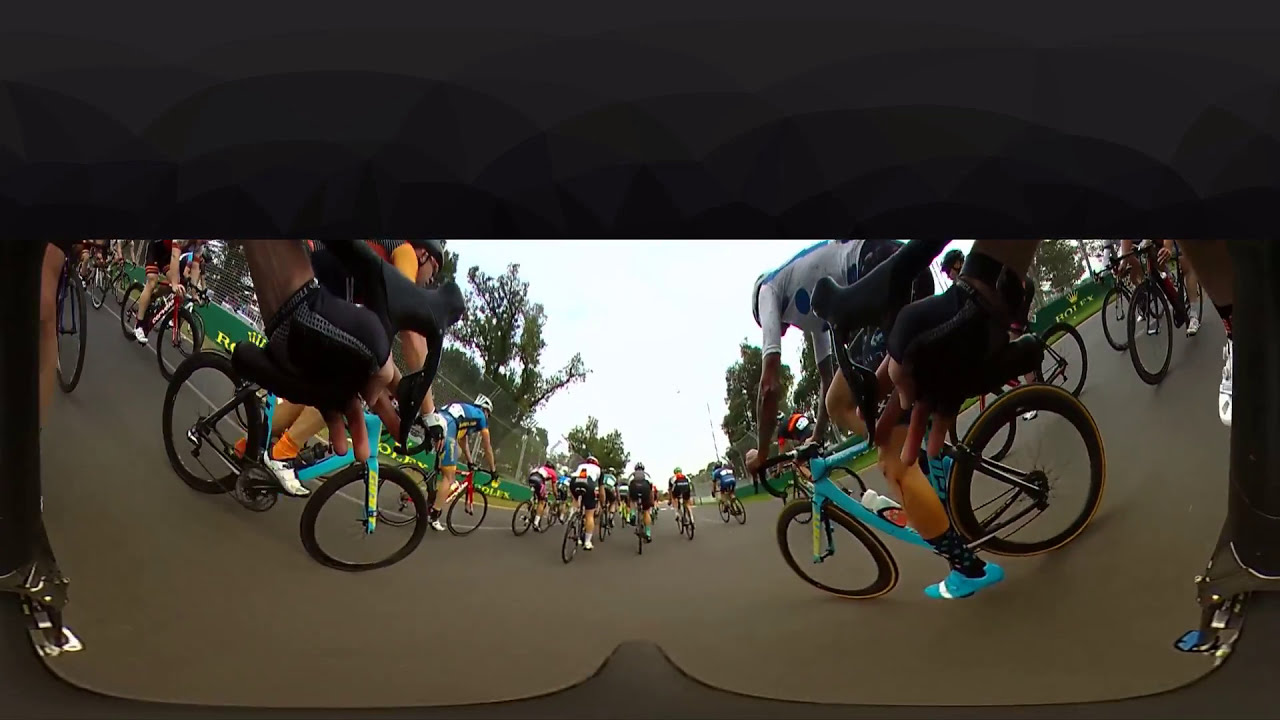This creatively taken photograph captures a dynamic bike race on a smooth, outdoor concrete road. The image employs a dual fisheye lens effect, creating two mirrored, slightly distorted views merged in the center, reminiscent of reflections on a pair of mirrored sunglasses. The race features numerous cyclists, all wearing helmets, sports clothing, gloves, and cycling gear, including multicolored jerseys, shorts, and shoes. The vibrant array of bicycles adds a splash of color to the scene. The roadway is flanked by boundary boards adorned with various texts and logos, though not entirely readable, enhancing the competitive atmosphere. Tall trees line both sides of the road, providing a green backdrop against a white, clear daytime sky. The borders of the image are framed by a thick, straight grey boundary at the top, adding to the unique composition.